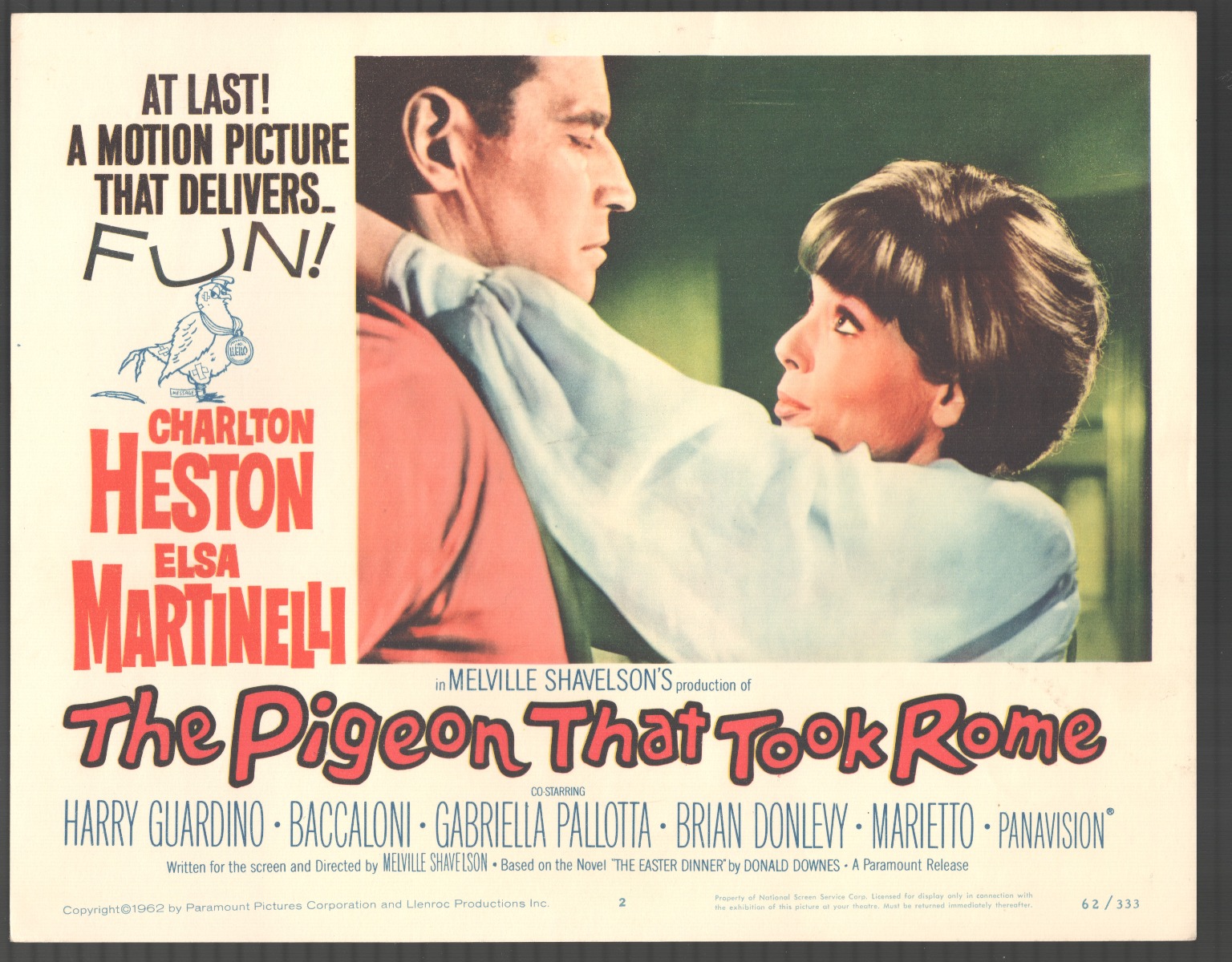This vibrant, vintage movie poster from the 1950s or 60s showcases an advertisement for the motion picture, "The Pigeon That Took Rome." The poster features a captivating full-color image, offset to the right, framed by a white background and a black border, which is slightly thicker on the right side. At the poster's center, a woman with short, wavy brown hair and a white sweater gazes up at a taller man she is embracing. The man's face is tilted down towards her, his eyes closed, and he wears a red shirt, though the top of his head is cropped out of the image. 

The background of the image depicts a green door and walls, adding depth to the scene. Surrounding the picture, text in various colors provides details about the film. On the left side of the poster, in brown writing, it reads, "At last a motion picture that delivers fun!" Below this text, a small blue sketch of a pigeon is displayed. Further down in red writing, the names "Charlton Heston" and "Elsa Martinelli" are prominently featured, along with the film's title, "The Pigeon That Took Rome," in bold letters. Smaller blue text above the title credits Melville Shavelson as the producer, and additional cast names such as Harry Guardino, Baccaloni, Gabriella Pallotta, Brian Donlevy, and Marietto appear at the bottom, emphasizing “Panavision” technology.